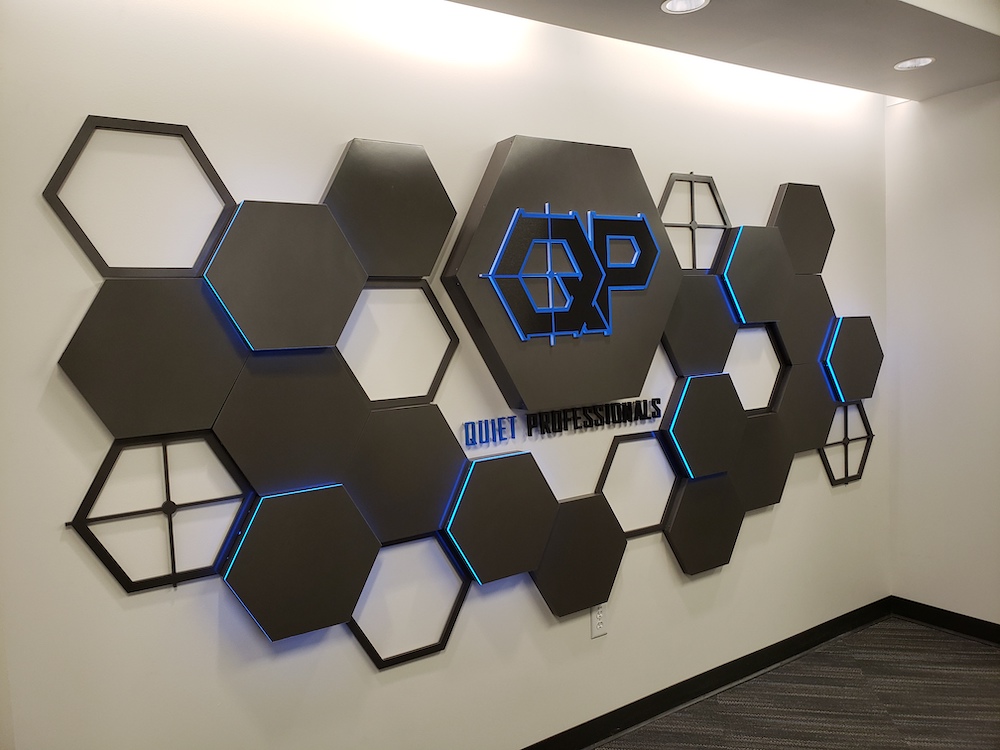This is a detailed color photograph capturing the entryway to a business featuring a distinctive logo art installation on a white wall with a slight drop ceiling and spotlights. The floor is covered with gray carpet bordered in black. The focal point of the image is an elaborate arrangement of hexagonal tiles forming a pattern across the wall. Some of these hexagons are solid black, some are hollow, and others have a crosshairs design in the middle. In the center of this installation, there is a larger black hexagon with the letters "QP" outlined in bright blue. Below it, in blue capital letters, the text "Quiet Professionals" is displayed. You can also see a partial view of the floor and an adjacent wall on the right edge of the image.